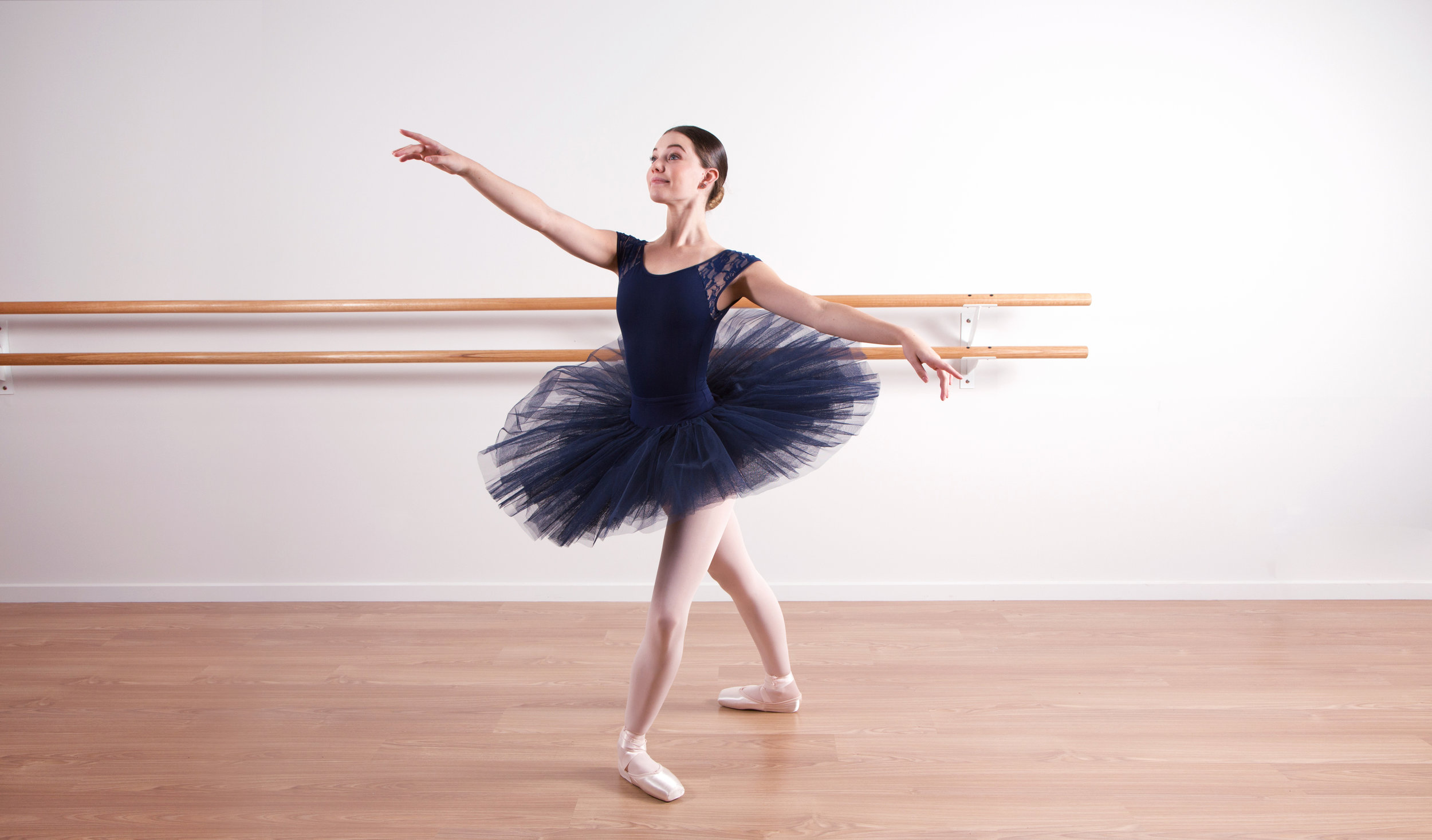This indoor photograph captures a Caucasian ballerina in a dance studio. She is poised gracefully in a ballet position, radiating pride. The ballerina wears a dark navy blue tutu, white tights, and white ballet shoes. Her short black hair is styled in a bun. Her left leg is extended forward and slightly to the right, while her right leg remains firmly planted, facing left. Her left arm, seen on the right side of the image, is stretched behind her, and her right arm, seen on the left, extends in front. The dance studio features a smooth hardwood floor and white walls adorned with brown wooden railings, indicative of a professional practice space.